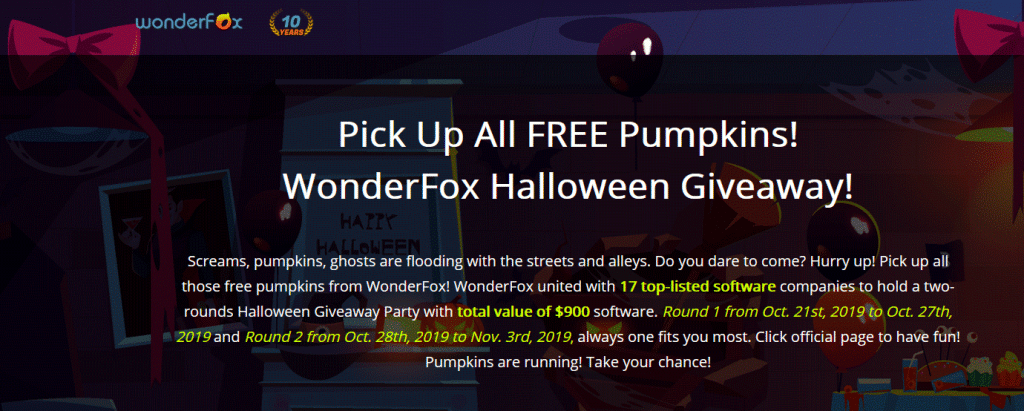**WonderFox Halloween Giveaway Promotional Banner: 10th Anniversary Celebration**

The promotional banner for the WonderFox Halloween Giveaway is richly designed to reflect a festive Halloween theme, using vibrant and spooky colors. Dominating the top left corner is the WonderFox logo, prominently displayed alongside a special badge marking their 10-year anniversary.

The main bold text commands attention, reading: "Pick up all free pumpkins, WonderFox Halloween Giveaway." Just below this, a tantalizing teaser follows: "Screams, pumpkins, ghosts are flooding the streets and alleys. Do you dare to come? Hurry up. Pick up all those free pumpkins from WonderFox." This sets a thrilling and eerie tone for the event.

The banner informs participants that the giveaway features contributions from 17 top-listed software companies. It unfolds in two rounds: the first from October 21, 2019, to October 27, 2019, and the second from October 28, 2019, to November 3, 2019. The total value of the software up for grabs is a staggering $900. 

The text prompts participants to click through to the official page to join the fun, with an enticing reminder that "pumpkins are running, take your chance." The background of the banner is richly illustrated with traditional Halloween imagery such as pumpkins and ghosts, rendered in dark, moody colors to heighten the festive ambiance.

Overall, this promotional banner effectively uses festive Halloween imagery and vibrant colors to attract attention and encourage participation in the WonderFox Halloween Giveaway, providing clear, engaging details about the event.